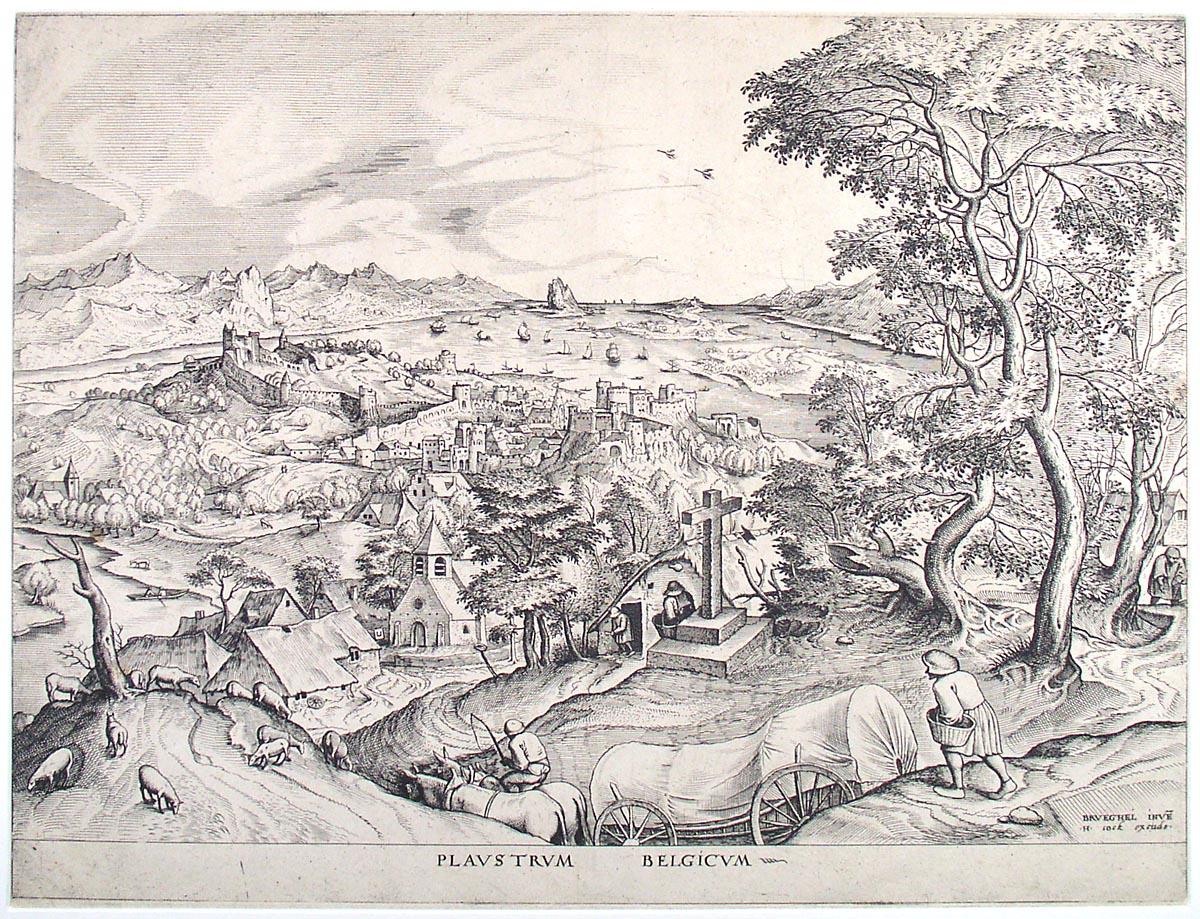This detailed black and white drawing, likely created with pencil or ink, depicts a serene country village scene from a hilltop overlooking a valley. The artist has illustrated a variety of elements in the foreground and background to create a rich tableau. In the foreground, a large stone cross stands prominently on the hillside, near a woman wearing a skirt and holding a basket, who is positioned as if overseeing the entire valley. Below her, we see a covered wagon drawn by two horses, with a man driving them and another person walking behind. 

The valley itself is filled with the tops of various building structures, dominated by a church with a steeple appearing in the center left. Off to the lower left corner, various animals such as cattle or perhaps sheep graze peacefully. The right side of the drawing is framed by several tall, leafy trees. 

In the background, a range of low mountains with what appears to be a castle or similar structure can be seen, with a few ships dotting the waters. Two birds are faintly visible in the distant sky, which is subtly shaded to indicate clouds. There's additional detail in the form of writing across the bottom of the drawing, which appears to be in Latin, reading "P-L-A-V-S-T-R-V-M-B-E-L-G-I-C-V-M." Despite the lack of color, the artist has managed to incorporate significant detail to bring this pastoral scene to life.